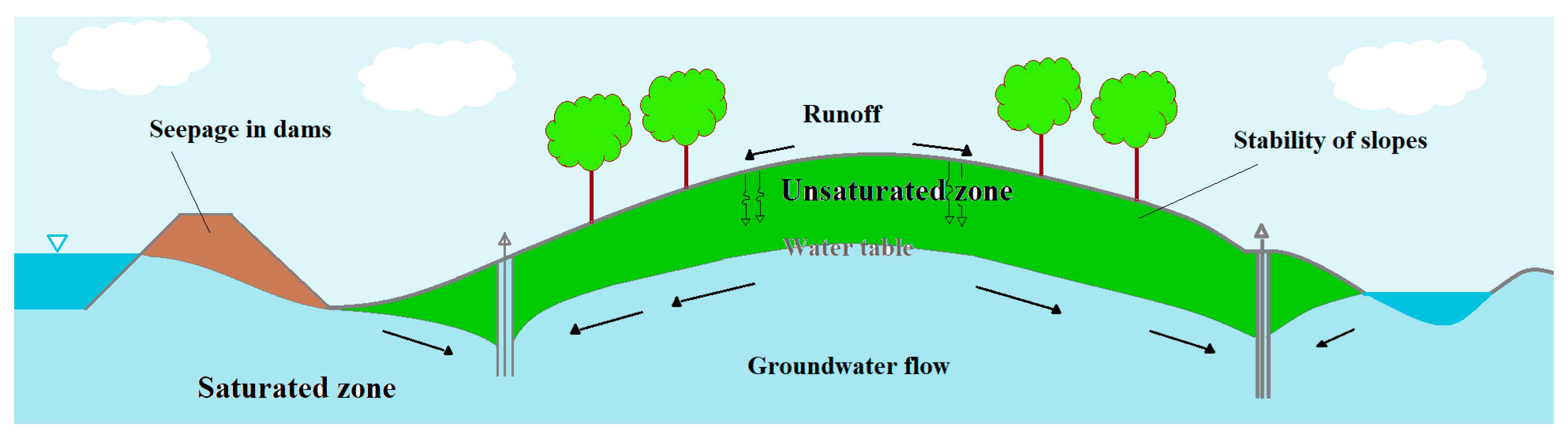This detailed illustration, likely intended for a book or brochure, depicts the mechanisms of groundwater flow and seepage. At the left, a brown trapezoid labeled "seepage in dams" extends upward, adjacent to a body of water resembling a lake or reservoir being held back. Below this trapezoid is a blue area marked "saturated zone," with an arrow indicating water movement towards the lower right.

Dominating the center of the image is a green hilly area signifying the "unsaturated zone," topped with grass and trees. Arrows labeled "runoff" point away from the crest of this hill, indicating surface water flow. The water table is delineated by a line separating the unsaturated zone above from the groundwater flow below, depicted with blue coloring and bi-directional arrows.

To the right, the illustration emphasizes "stability of slopes," with an arrow pointing to the unsaturated zone's right section, where another depression contains some water. Above the entire scene, a blue sky with clouds provides a backdrop, reinforcing the image's focus on environmental and hydrological processes.